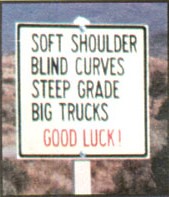The image features a road sign with a bold, black border. The sign itself is white and prominently displays various warnings in black, capitalized text across several lines. The warnings read: "SOFT SHOULDER," "BLIND CURVES," "STEEP GRADE," and "BIG TRUCKS." At the bottom of the sign, in a striking pink text also in capital letters, is the phrase "GOOD LUCK!" followed by an exclamation mark. This sign is mounted on a white post, visible both at the top with a small nub and extending downwards to the bottom of the image. The background showcases a scenic landscape of rolling hills, transitioning from bluish-gray at the top to a more brownish beige near the bottom. The hills are sporadically dotted with green shrubbery and foliage, adding a touch of color to the predominantly earthy tones.